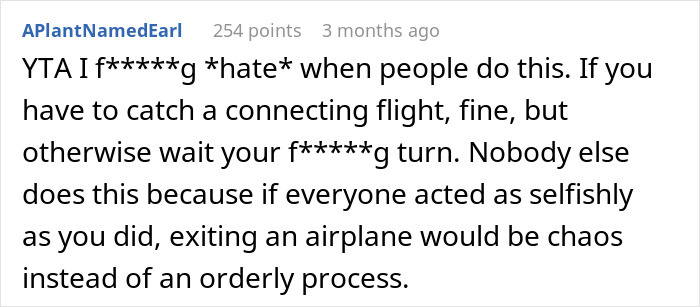This image is a cropped screenshot from Reddit, either from the app or the website. It is a small excerpt focusing on a single comment bordered by a light grey outline. The comment's author uses the username "A Plant Named Earl," displayed in blue font with each word capitalized and the rest in lowercase letters. This particular comment has received 254 points and was posted three months ago. 

In the comment, the user expresses frustration towards another user with the acronym "YTA" (You're the Asshole), a common verdict in Reddit's 'Am I the Asshole?' community. The comment reads: "YTA, I ****** hate when people do this. If you have to catch a connecting flight, fine, but otherwise wait your ****** turn. Nobody else does this because if everyone acted as selfishly as you did, exiting an airplane would be chaos instead of an orderly process." The comment contains censored swear words, replaced with asterisks, reflecting the author's strong disapproval of the behavior described.